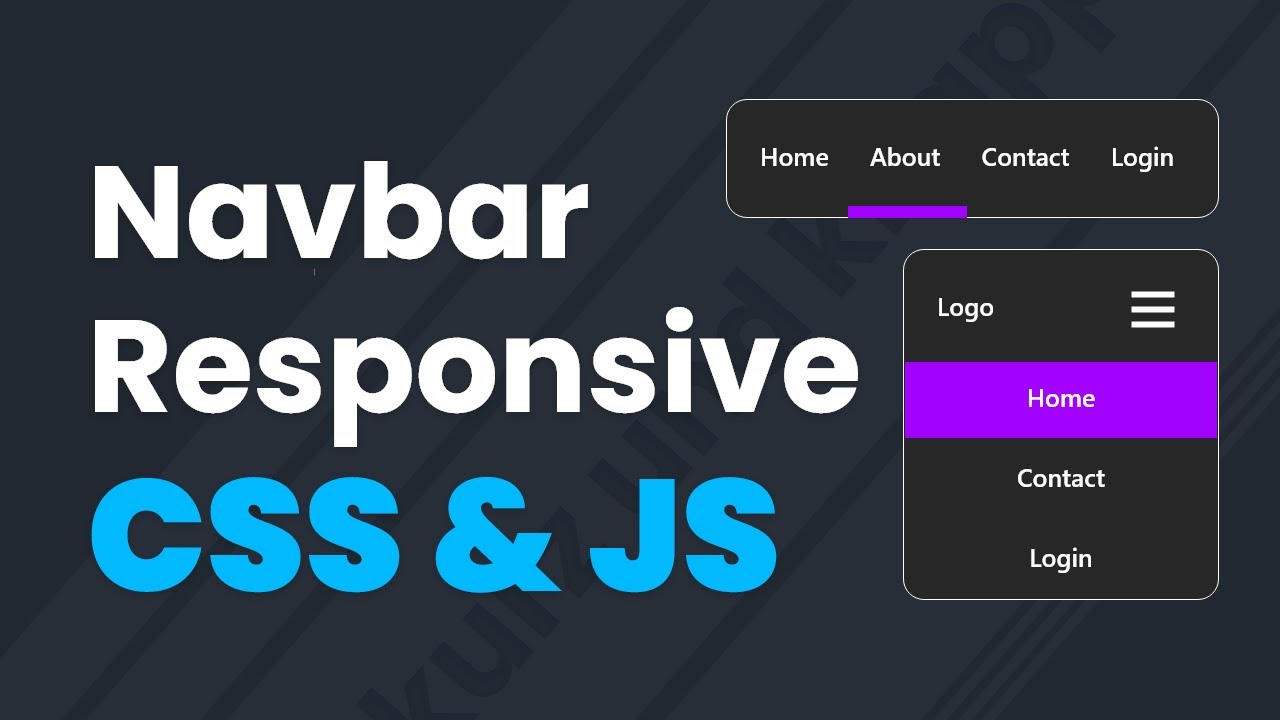The image depicts a user interface design mockup with a dark background. Visible through the dark backdrop is a hint of some printed material in the background. In the upper left-hand corner, white text reads "Nav Bar Responsive." Adjacent to it in blue text are the letters "CSS" and the ampersand symbol, followed by the letters "JS" also in blue.

On the right side, there is a sleek, black rectangular button with curved edges, highlighted by a silver, shiny metallic border. Inside this button, white text reads "Home," "About," "Contact," and "Login," with the word "About" underlined by a purple line. 

In the lower right-hand corner of the image, there's a wider black rectangle with a chrome finish around its edges. At the top of this rectangle, the text "Logo" is displayed. Below it, there are the words "Home," "Contact," and "Login," with "Home" featured in a purple rectangle.

This design mockup illustrates a modern, responsive navigation interface with emphasis on simplicity and visual appeal through the usage of contrasting colors and sleek metallic accents.